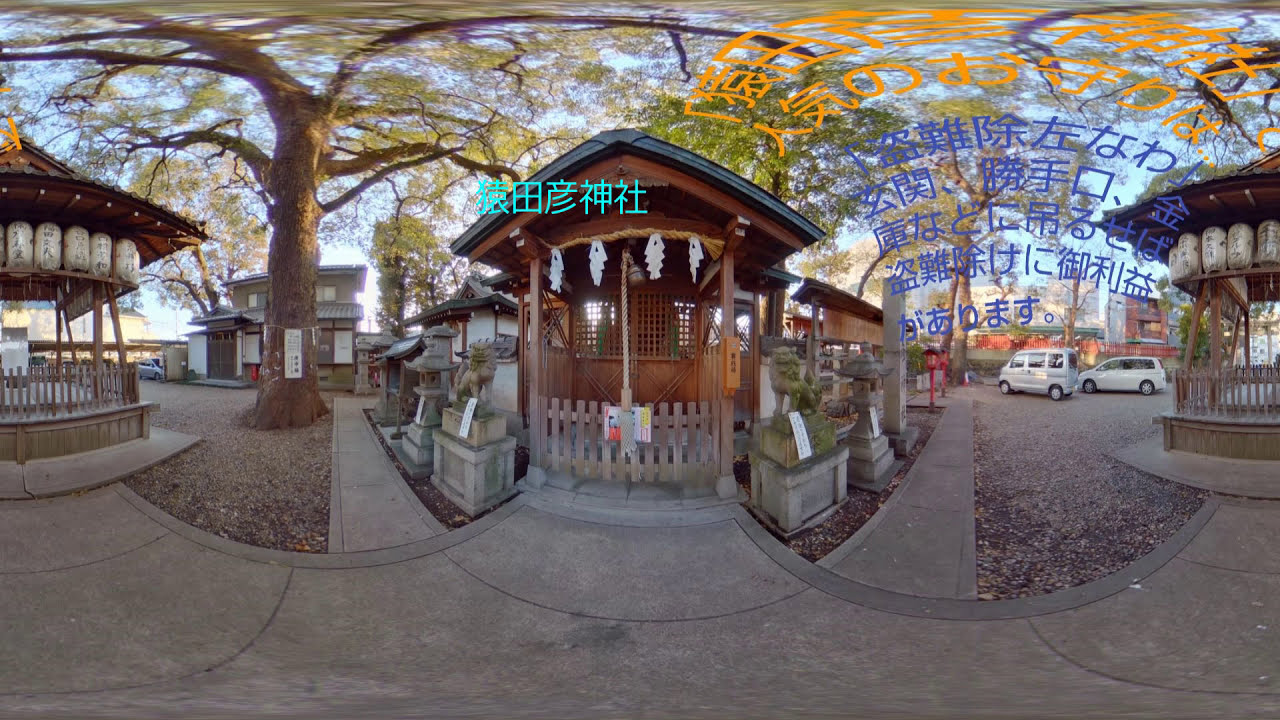The image, likely captured by a fisheye security camera, depicts an outdoor scene of a traditional Asian market or potentially a monastery. The architectural style, featuring oriental elements such as kiosks with wooden frames and greenish roofs, conveys a distinctly Asian aesthetic. The lower section reveals a gray sidewalk extending into the background, intersecting with a tree whose branches canopy the upper part of the image, adding a natural touch to the setting.

Central to the scene, a pagoda-like structure with a wooden picket gate and lattice doorway stands prominently. Statues and lanterns, possibly Chinese or Japanese, flank this area, adding cultural richness. Various Asian characters in green, blue, teal, yellow, and orange adorn the image, hinting at signage or decorative text. To the right, a few white cars are parked, offering a modern contrast to the traditional elements.

The scene is set under a clear, blue sky, with just a hint of sunlight casting shadows, suggesting it's either late evening or early morning. The market or monastery appears serene and devoid of people, emphasizing its tranquil atmosphere and timeless beauty.